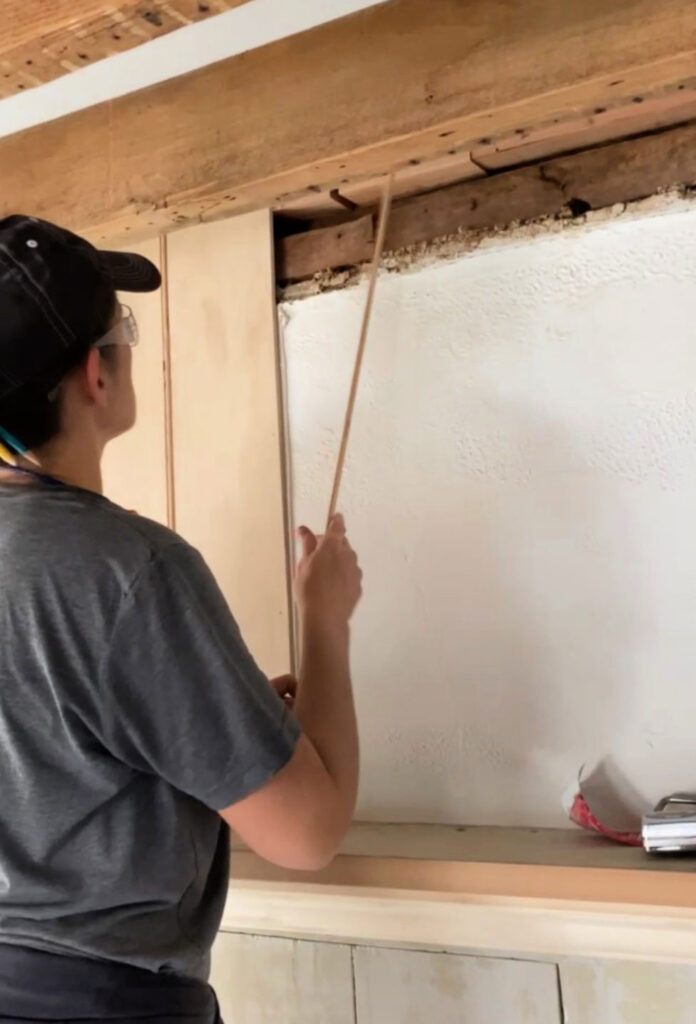In this image, a person is positioned on the left side, wearing a black cap, clear safety glasses, a gray shirt, and gray pants. They are holding a gray t-shirt in one hand and a brown stick in the other, extending the stick towards several plates situated just below what appears to be an opening of a window. Above this area, there is a brown section of ceiling followed by a white strip, with a brown beam crossing horizontally.

Towards the left, light gray slats descend vertically. In the foreground, a white wall, possibly made of cement, stands with a section of brown wood just above it. The window sill is made of brown wood, and beneath it is a white piece that resembles a frame. Below the sill, there are off-white tiles.

On the right side of the image, there is a small gray box, with an unidentified pink object located right next to it.